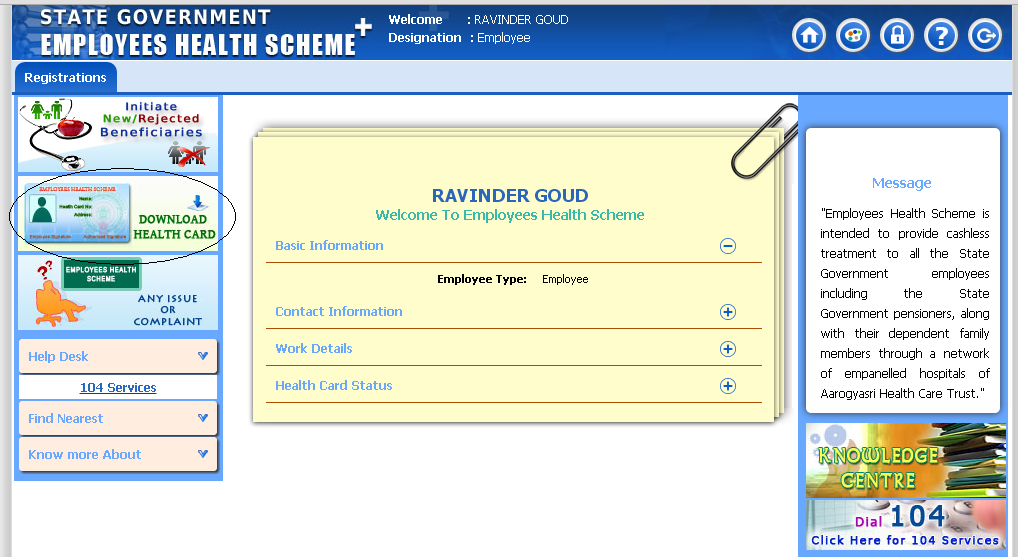**Caption: Detailed Overview of State Government Employee Health Scheme Webpage**

The webpage is a portal for the State Government Employees Health Scheme. In the top left corner, the title "State Government Employees Health Scheme" is prominently displayed. Below this, the user is greeted with the message "Welcome, Ravinder Goode," along with the designation "Employee."

The left-hand column features a series of sections. The first section, titled "Registrations," contains an icon of a stethoscope paired with an apple and the text "Initiate New/Rejected Beneficiaries." Adjacent to this is another icon depicting a family with a red 'X' over it, indicating the initiation process for new or rejected beneficiaries.

Following this, there's an area bordered by a black oval shape that includes an icon of an identification card. Beside this icon, the text reads "Download Health Card." Below this icon, another segment titled "Employee Health Scheme" includes an image of a person with two question marks above their head, accompanied by the text "Any Issue or Complaint."

Further down, the section titled "Help Desk 104 Services" provides additional information with options like "Find Nearest" and "Know More About."

In the center of the page, a more personalized greeting appears: "Ravinder Goode, welcome to Employee Health Scheme." This section includes "Basic Information," details about "Employee Type," "Employee Contact Information," "Work Details," and "Health Card Status."

The right-hand column starts with a message that defines the scheme. It reads, "Employees Health Scheme is intended to provide cashless treatment to all the state government employees, including state government pensioners, along with their dependent family members through a network of panel hospitals of Arogylossy Healthcare Trust."

Below this message, there is an image of a stack of books accompanied by the text "Knowledge Center." It also includes the information "Dial 104" and a clickable link "Click Here for 104 Services."

Overall, the webpage provides comprehensive data regarding the health scheme, offers a user-friendly interface for the employees, and provides easy access to various health-related services and support.